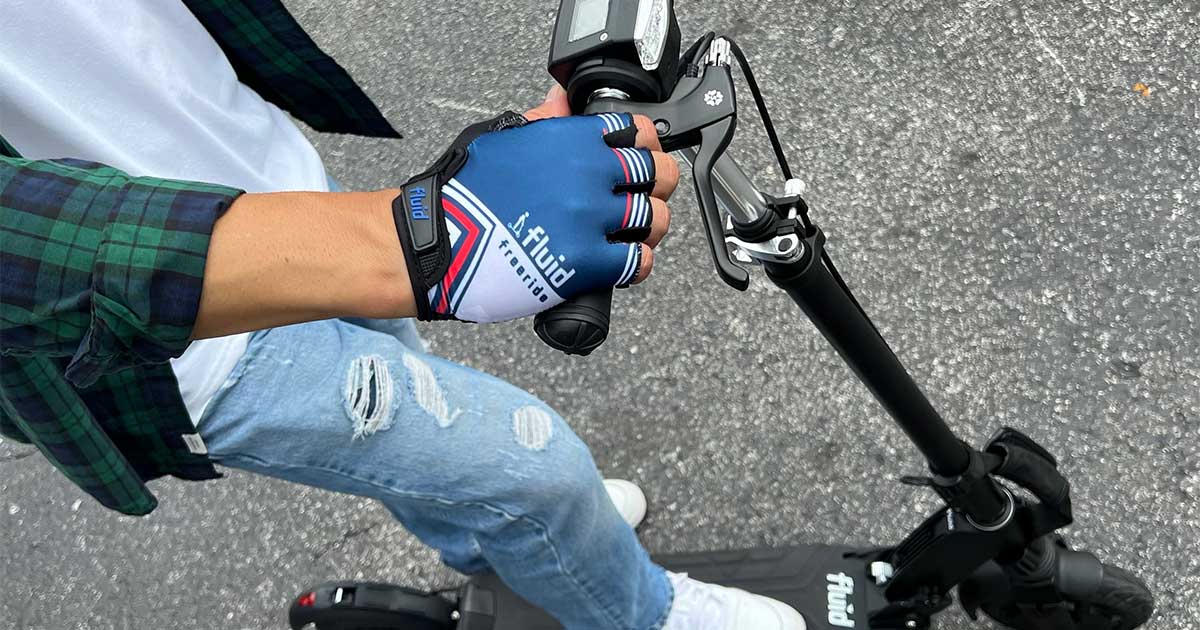In a sunlit outdoor scene, the image captures a downward view of a young man standing on a small, black kick scooter designed for one foot pushing. The concrete ground below is a speckled mix of gray and white, indicating a well-worn surface. The scooter, identifiable by its long black neck, flat black base, and tiny front wheel, features a throttle and a small display on the handlebar. 

The man, who appears to be Caucasian, has muscular arms and is fashionably dressed in ripped blue jeans with multiple holes, prominently one large tear on the right leg. He's clad in white tennis shoes and a white t-shirt, topped with an unbuttoned green and blue plaid shirt. On his right hand, he wears a blue and red fingerless glove, gripping the scooter's steering bar. Only his lower half and right arm are visible in the image, with his bent right knee planted firmly on the scooter. Despite the sunny weather, the lack of a prominent shadow suggests that the light is diffuse and not too harsh.